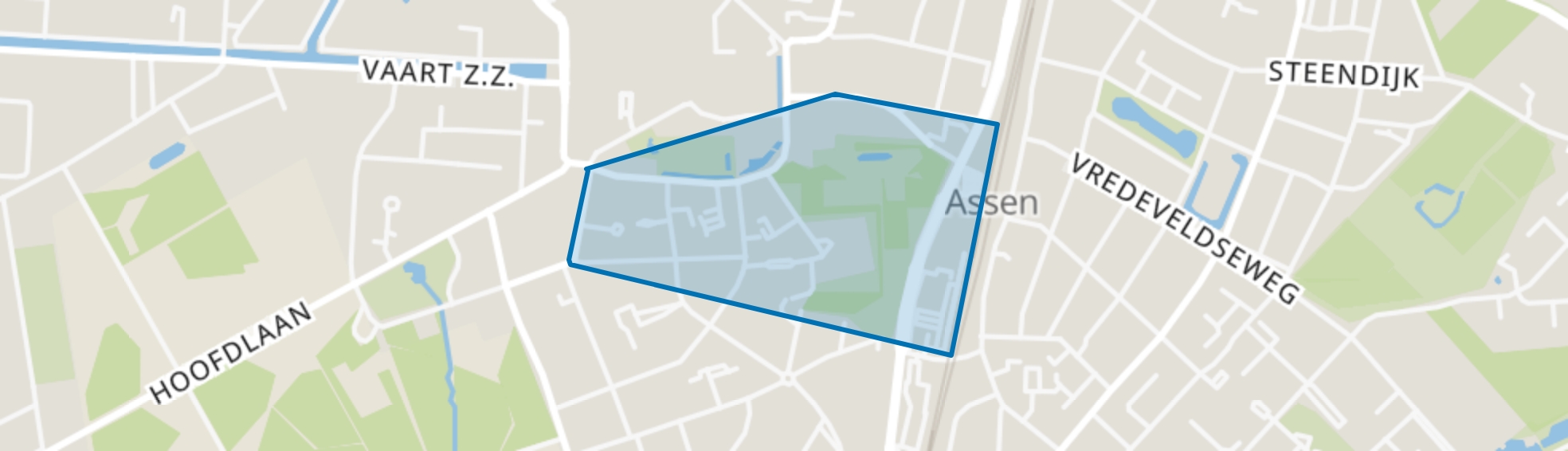The image displays a detailed map, likely of a European city, featuring several regions labeled with text in a foreign language, possibly Dutch. Key areas are identified as Hufblon, Bartz ZZ, Assen, Reveldzvig, and Steendvig, with alternate spellings including Hoeftelaan, Wart ZZ, Steenedijk, and Redderveld. The map is primarily composed of colors such as tan, white, blue, black, green, olive green, and light beige. Central to the map is a highlighted area in blue, likely indicating a significant region or waterway. The map also includes a network of white lines representing roads and green patches that might denote parks. The overall appearance is akin to an ordinary internet map utilized for navigation or direction-finding purposes.